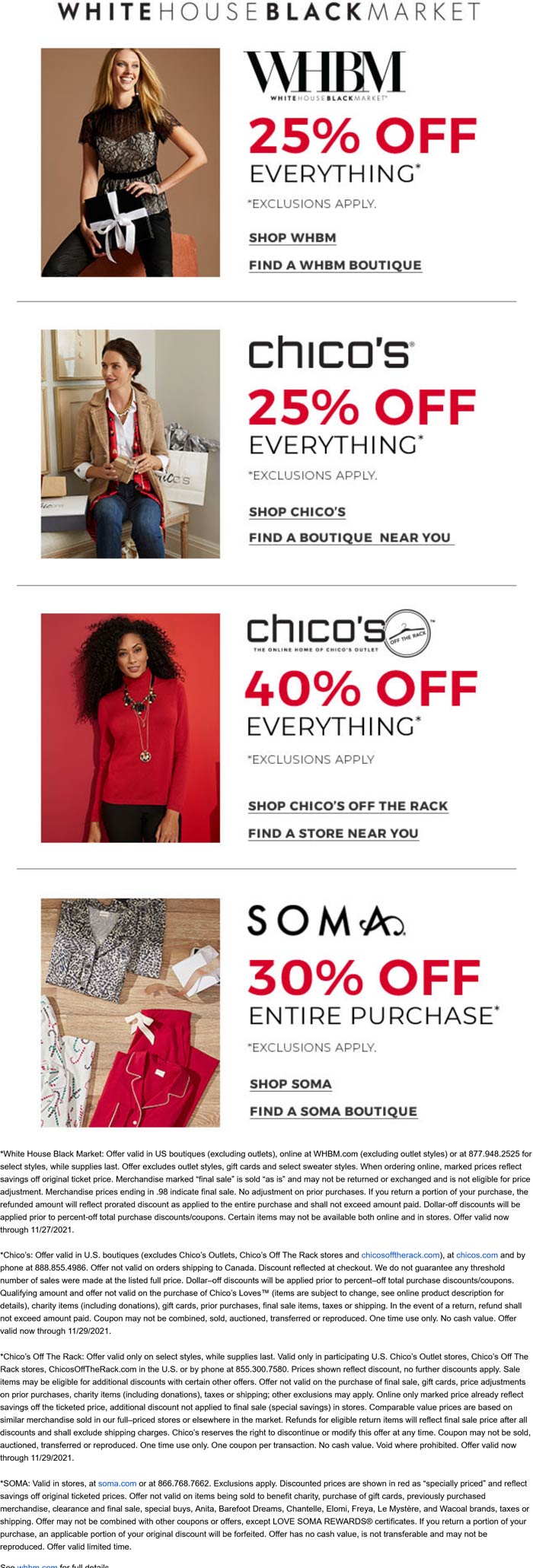The image is a vertical, portrait-oriented screenshot likely taken from a mobile phone app. The screenshot itself, set against a white background, prominently displays a series of clickable advertisements for various fashion retailers. At the very top, the title "White House Black Market" is divided into two font colors: "White" and "Black" in black, and "House" and "Market" in grey.

Below the title are four horizontally aligned thumbnails, each separated by thin grey borders. The first thumbnail features the abbreviation "WHBM" alongside an image of a Caucasian woman with blonde hair, dressed in a black shirt and black pants, with a red text that declares "25% off everything."

The second thumbnail showcases another Caucasian woman with black hair, wearing a brown jacket over a white and red shirt and blue jeans. This image is labeled "Chico's" and highlights "25% off everything" in red.

In the third thumbnail, an African American woman with thick black hair can be seen wearing a red sweater and black pants. This segment, also labeled "Chico's," advertises "40% off everything" in red font.

The fourth and final thumbnail displays a collection of clothing items spread out on a wooden floor, with the label "Soma" and an offer of "30% off entire purchase" written in red.

Beneath these thumbnails, the screenshot includes four paragraphs of text in black font on the white background, although the font size is too small to be legible.

Overall, the image encapsulates a series of promotional offers from different fashion brands, all prominently displaying sale information in red to catch the viewer's attention.